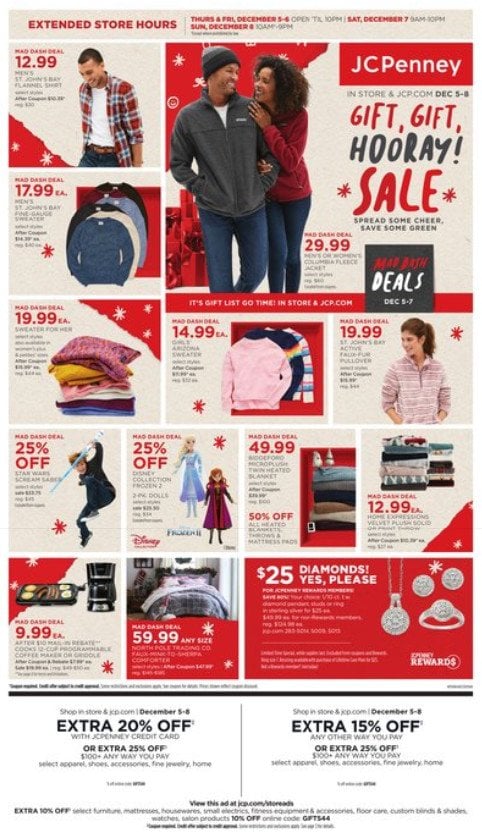The image appears to be a holiday-themed newspaper style ad for JCPenney, likely sourced from their website. The ad prominently features a festive color scheme with red highlights and white snowflakes. At the very top, in bold red lettering, the ad announces extended store hours: Thursday and Friday, December 5th and 6th; Saturday, December 7th from 9 a.m. to 10 p.m.; and Sunday, December 8th from 10 a.m. to 9 p.m.

The layout is divided into approximately thirteen sections. In the upper left corner, there's an image of a light brown-skinned male wearing an unbuttoned plaid shirt over a white T-shirt, which advertises a "Mad Dash Deal" for $12.99. Beneath the main JCPenney heading, we see a couple who appear to be Black: the woman has curly brown hair, and the man sports a beanie and a gray zip-up fleece. Both are dressed in blue jeans. This section promotes a "Gift, Gift, Hooray Sale" with items priced at $29.99.

Moving through the ad, there are additional "Mad Dash Deals," including sweaters priced at $17.99 in various colors such as blue, black, and white. Another deal features multicolored sweaters, including a mustard yellow one, seemingly targeted at mothers. A young white female models a pinkish-gray zip-up sweater in another promotional section.

Towards the bottom of the ad, there is a "Mad Dash Deal" for 25% off select items. This section is illustrated with an image of a young boy, around 12 or 13 years old, energetically playing with what appears to be a toy lightsaber from Star Wars. Adjacent to this, there are Disney Frozen-themed dolls available for 25% off. Bedding sets are listed at $59, and there's a mention of "$25 diamonds" as part of a special reward offer.

Finally, the bottom part of the ad features numerous coupons offering additional discounts: 25%, 20%, and 15% off various purchases, accompanied by detailed terms and conditions.